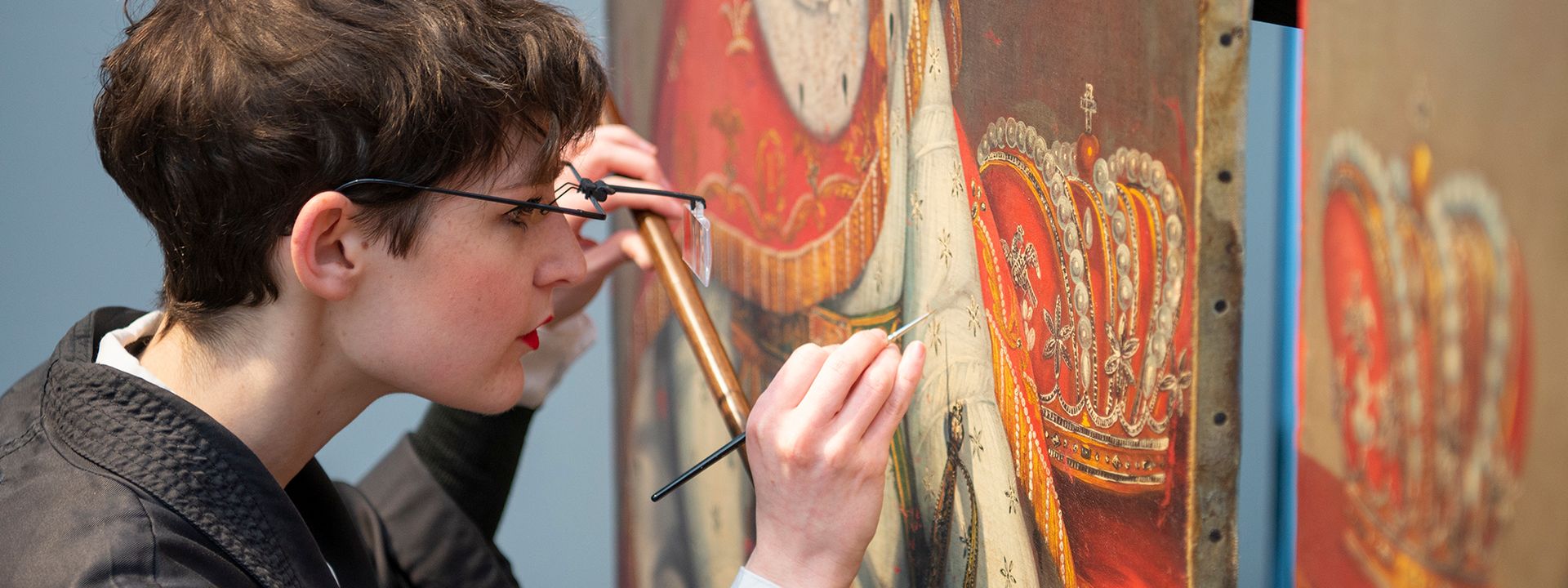A woman artist with short, stylish black or brown hair, dressed in a black coat over a long-sleeve black shirt, is meticulously restoring an old painting. She is positioned to the left of the canvas, concentrating intensely through a pair of specialized magnifying glasses designed for detailed work. She is applying retouches to a red royal crown within the painting, suggesting a regal subject. In her right hand, she uses a very thin black paintbrush, and in her left hand, she steadies herself with a light brown measuring tool. The background features light blue walls, which emphasize the contrast and focus on her precise, delicate technique. The artist's workspace and careful attention to detail create an atmosphere reminiscent of a museum restoration project.